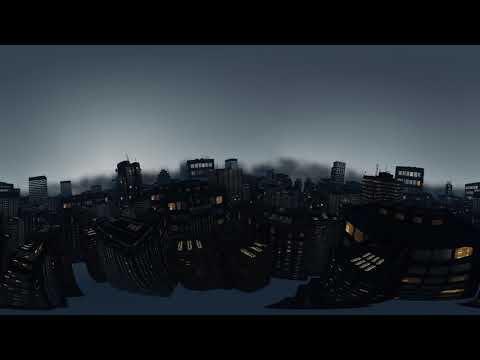This image, either a computer-generated illustration or a photograph, showcases a nocturnal cityscape framed by solid black borders on the top and bottom. The central focus is a skyline composed of various black buildings, with some displaying small yellowish-white illuminated windows, hinting at nighttime or just after sunset. The dark gray sky above transitions to a slightly lighter hue towards the horizon, suggesting a fading twilight. Below the skyline, there appears to be a body of water with reflections of the buildings and small white boats interspersed around. The overall palette of the image consists of predominantly dark tones, including dark blue and gray, giving the scene a somewhat somber and blurred aesthetic.